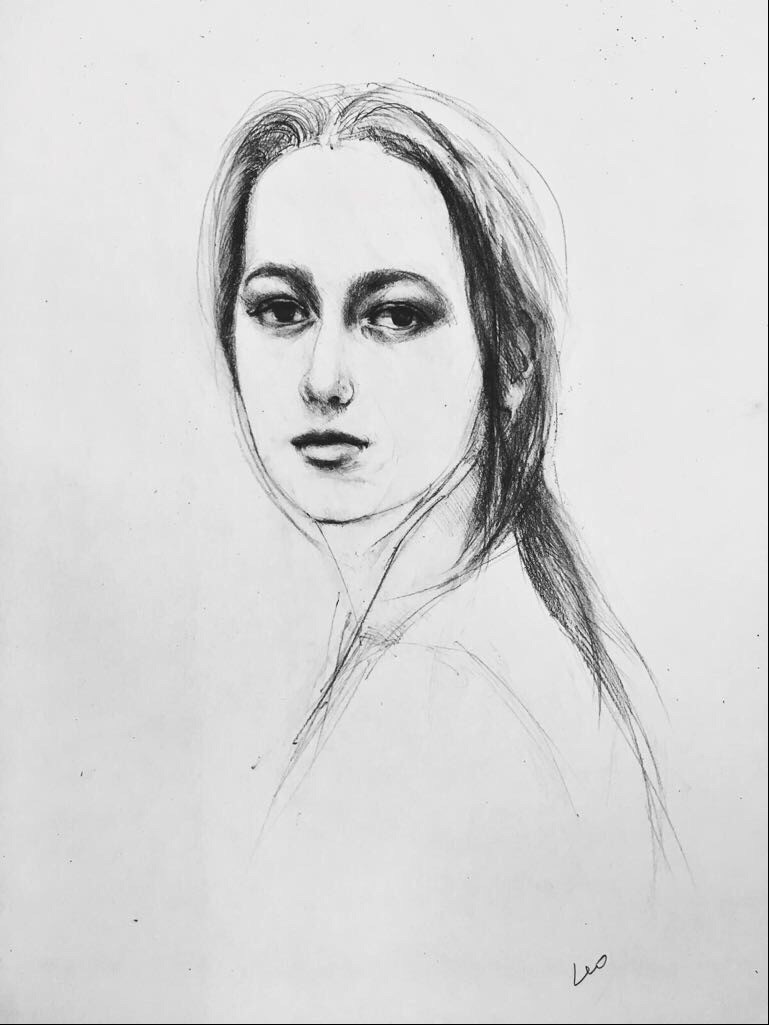This exquisite charcoal sketch, rendered on a slightly vertical sheet of paper, captures the nuanced beauty of a young woman. Her body is gracefully oriented towards the left, while her head is turned to gaze over her left shoulder, directly engaging the viewer with her dark, captivating eyes. The intricate detailing around her eyes, including the expertly shaded eye sockets, eyelids, and the medium-thick eyebrows, adds depth and realism to her expression. Her long hair cascades gracefully, framing her narrow nose and delicate features. The artist, Leo, has masterfully employed shadowing and texture to bring this evocative portrait to life.